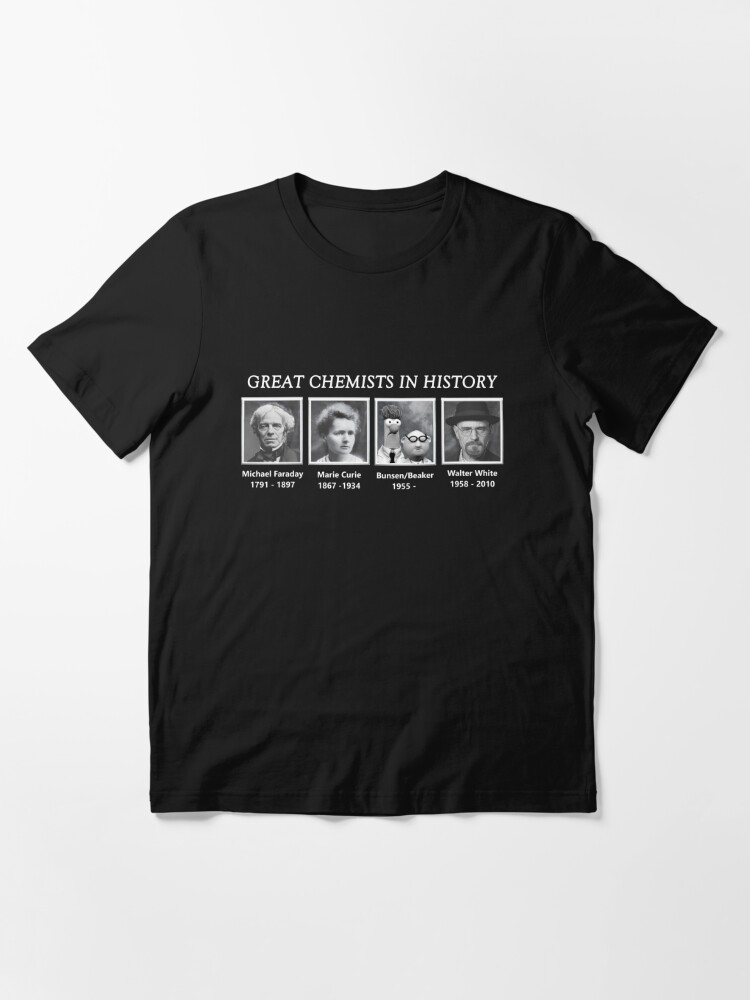The image displays a black cotton t-shirt with a crew neck and short sleeves, laid flat against a stark white background. Centered prominently in the middle of the t-shirt is the text "GREAT CHEMISTS IN HISTORY" in white, capital letters. Below this inscription, four images are neatly arranged in a row from left to right. The first image is labeled "Michael Faraday, 1791 to 1897," depicting an older gentleman. The second image shows "Marie Curie, 1867 to 1934," accompanied by an illustration of her. The third set of images features cartoon characters labeled "Bunsen Beaker, 1955 onward." Finally, the fourth image portrays "Walter White, 1958 to 2010," showing a man wearing a black top hat. The t-shirt's setting and style suggest it is a humorous take on historical chemists, combining real and fictional characters to create an amusing homage.